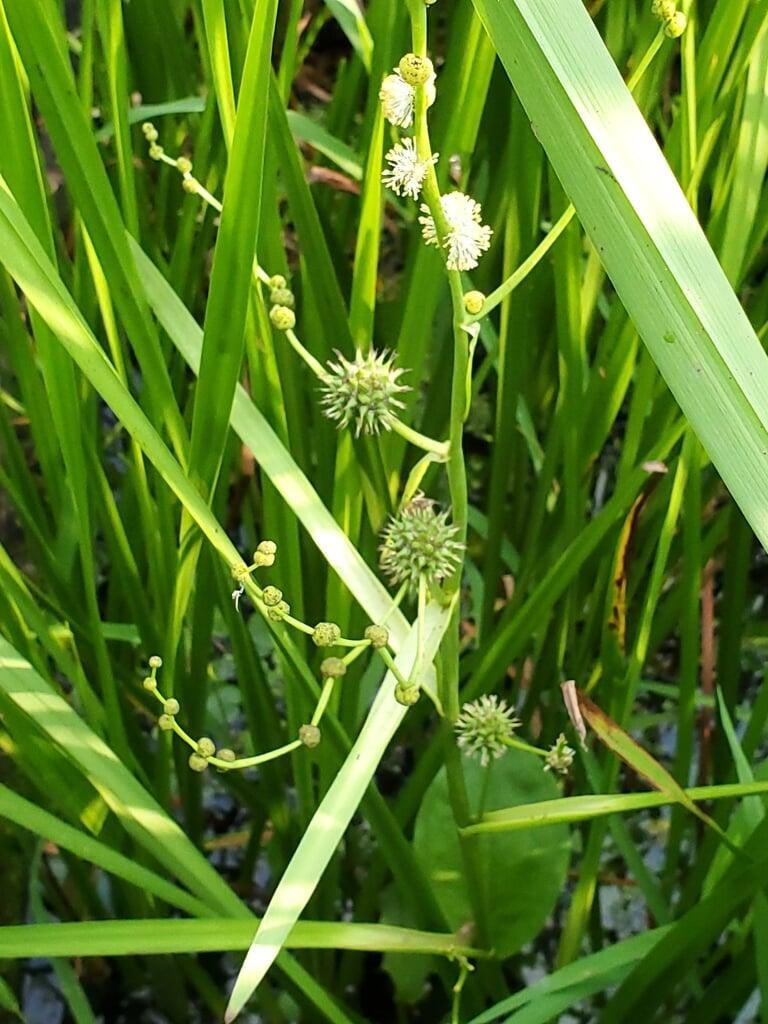This image captures a detailed, close-up view of a lush, green marsh area, featuring a dense array of tall grass blades. Dominating the center is a single, thicker plant starting from the bottom and extending upwards, adorned with spiky white flower projections at the top and green spiky projections beneath. Additional elements include small green ovoid balls climbing around the stem, likely to develop into the larger spiky structures. The ground beneath appears wet, suggesting a marsh or swamp environment, with water reflections contributing to the scene's vibrancy. Scattered throughout are vivid green and some yellowing or browning blades of grass, emphasizing the thriving yet slightly varying plant life within this marshy locale. A single oval leaf is partially visible toward the right center of the image, adding to the intricate details captured in this vibrant and close-focused photograph.